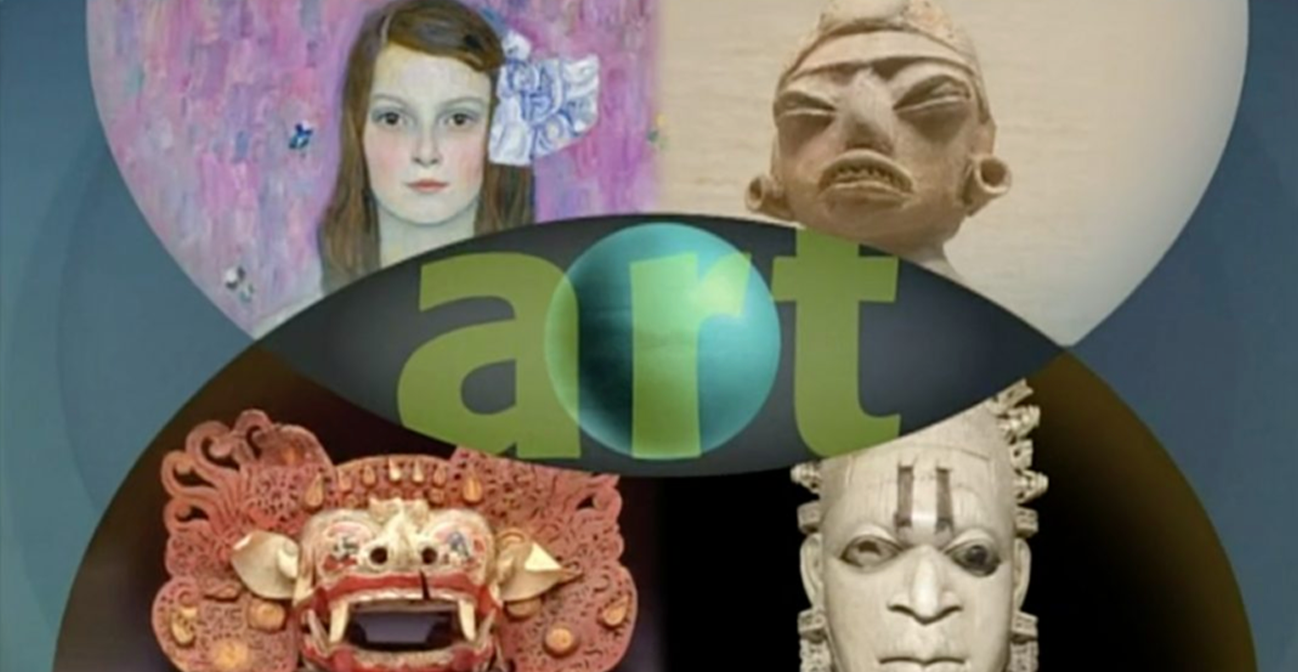The image, likely from a museum brochure, is a rectangular composition divided into four quadrants, each featuring a distinct piece of art. Dominating the center are two overlapping semi-circles, creating a Venn diagram effect with their intersection showcasing the word "art" in bold, grassy green letters. Notably, the 'R' in "art" is encapsulated within a sphere. The upper left quadrant presents a detailed color pencil illustration of a young girl with shoulder-length brown hair against a purple background, reflecting a Eurocentric style. In the upper right quadrant sits an ancient Mayan sculpture head, displaying intricate carvings. The lower left quadrant features an imposing Aztec or Mayan demon mask, exuding a sense of mysticism and history. The bottom right quadrant houses an oriental ivory carving, possibly from India, demonstrating fine craftsmanship. This curated selection of art pieces seems intended to represent a diverse array of cultural artifacts, suitable for both an art museum and a historical exhibition.